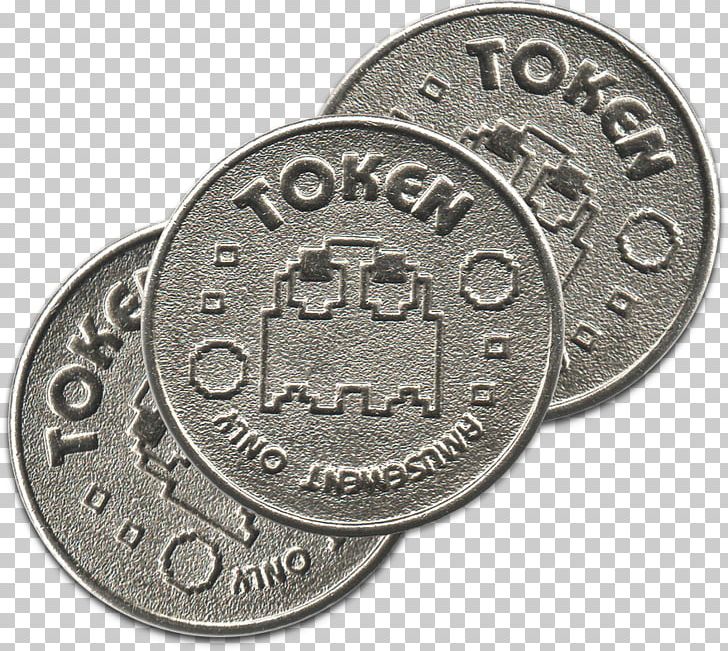The image displays three large arcade tokens prominently centered on a white and gray checkerboard background, indicating the intend to make the image translucent. The tokens, which are silver with shades of gray and black, are diagonally aligned from the bottom left to the top right corner. The middle token is fully visible and overlays the other two, which are partially obscured. Each token features bold, all-capital text: "TOKEN" at the top and "AMUSEMENT ONLY" at the bottom, with the latter being upside down. A cartoon image, possibly resembling a Pac-Man character or a squid, is centered on each token. The edges of the tokens are smooth yet raised, while the centers appear rough. This detailed depiction suggests the tokens are designed for use in an arcade setting or a similar amusement environment.